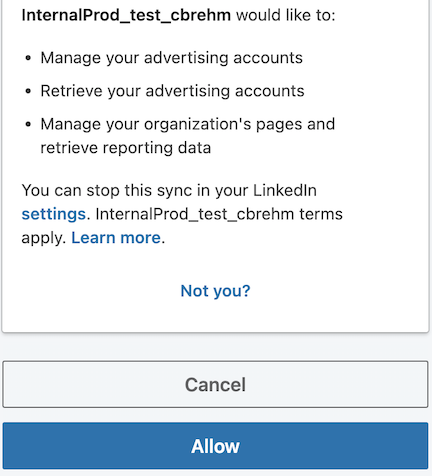A vertical screenshot, likely from a mobile app, displays a settings page. At the top, there is a white box with a subtle gray border containing text. The text begins in bold black with "internal_prod_test_CBREHM" and continues in less bold gray with "would like to:" followed by three bullet points:

1. Manage your advertising accounts.
2. Retrieve your advertising accounts.
3. Manage your organization's pages and retrieve reporting data.

An additional line states: "You can stop this sync in your LinkedIn settings." 

Beneath this list, it reads: "internal_prod_test_CBREHM terms apply. Learn more." and a blue "Not you?" link is present. At the bottom, there are two buttons: a gray "Cancel" button and a blue "Allow" button.